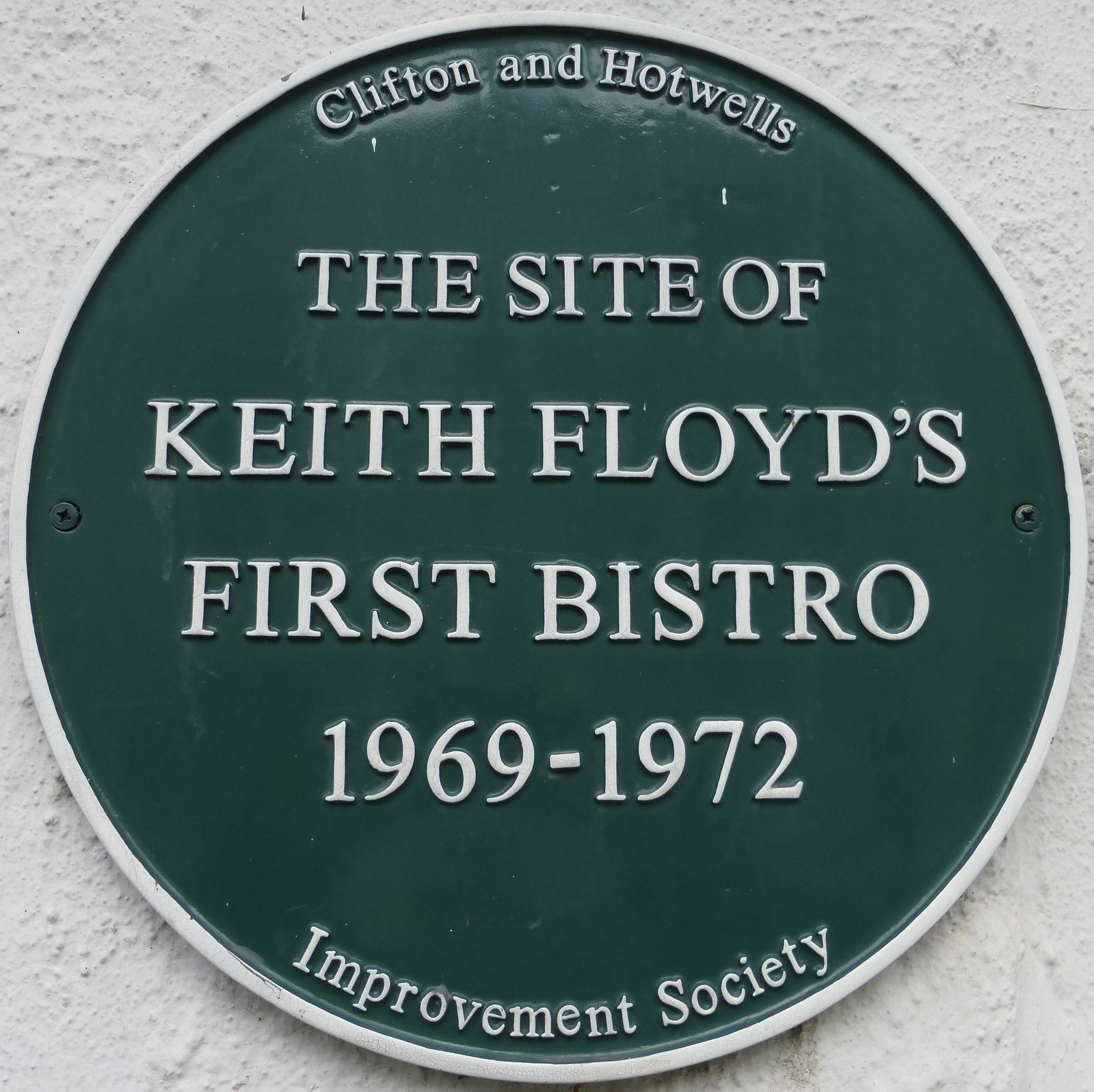The image shows a circular, dark green plaque mounted on a white-painted stone wall. The plaque features raised white lettering that reads, at the top, "Clifton and Hotwells," followed by "The site of Keith Floyd's first bistro, 1969-1972." Below that, it states "Improvement Society." The words "Clifton and Hotwells" are prominently capitalized in part, with "CLIFTON" and "HOTWELLS" in all caps. There are two visible screws securing the plaque, one on the far left and one on the far right. The green circle with white text contrasts sharply against the white square background, giving it the appearance of a large button or medallion on the wall.